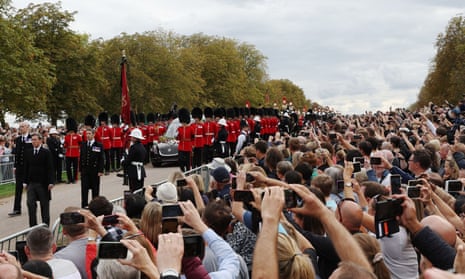The image captures a solemn procession, likely the funeral of Queen Elizabeth II, unfolding on a bustling street in England. The crowd, separated by silver barriers, is filled with thousands of spectators, all with their cell phones raised to capture the moment. In the center of the photograph is a black hearse, reminiscent of a limousine, flanked by the Queen's Guards. The guards are easily recognizable by their red jackets, black trousers, and iconic bearskin hats. In front of the hearse are four to five men in black suits, possibly family members or dignitaries, leading the vehicle along its route. The grandeur and somber atmosphere are palpable, as people pay their respects to the late monarch.